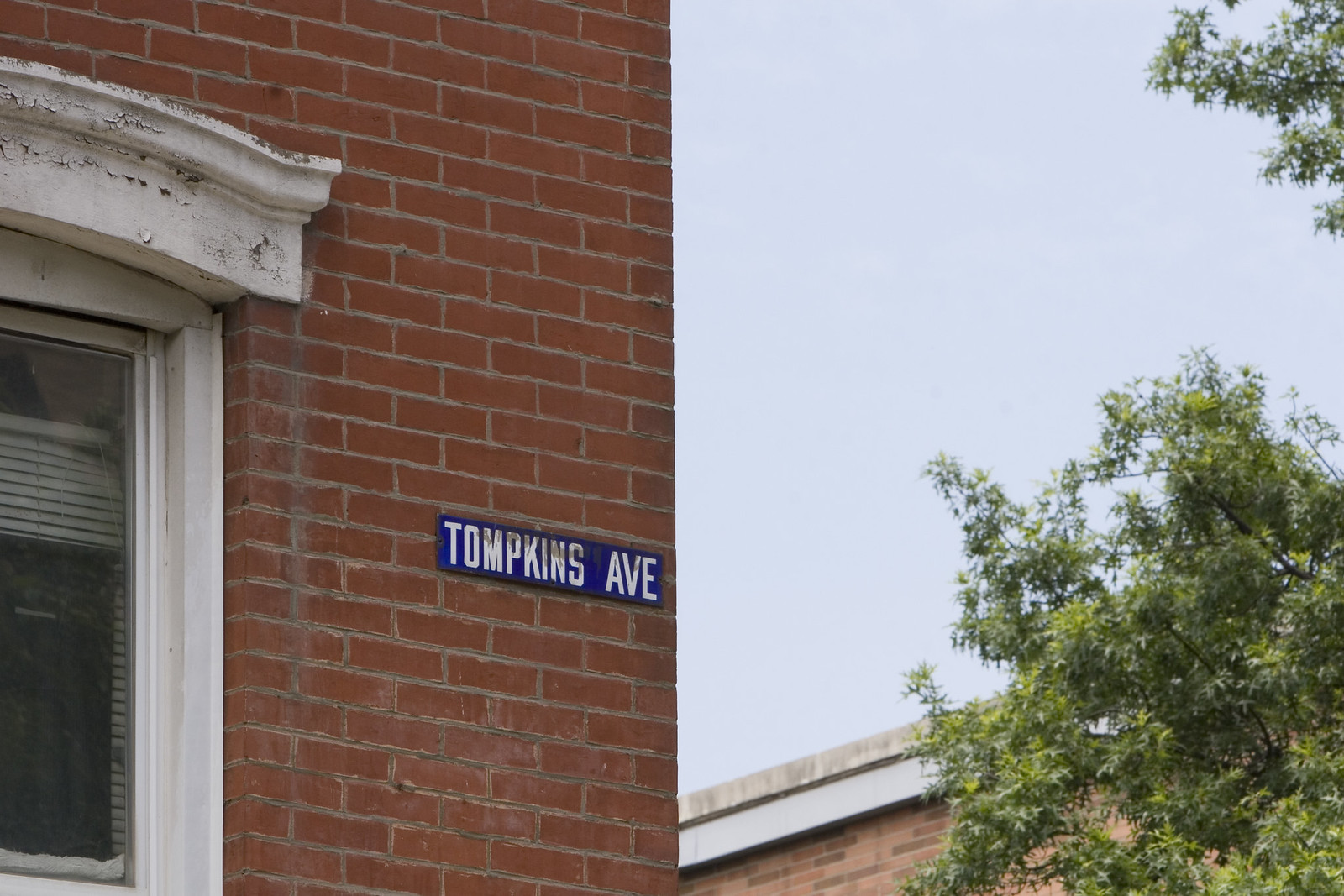This photograph, taken outdoors, captures the intricate details of an urban setting. Dominating the left side of the image is the rich, red-brown brick façade of a building. The bricks contrast sharply with the white window casing mid-frame, where a curved molding elegantly crowns the window. A bright blue street sign that reads "TOMPKINS AVE" in bold, white, all-capital letters is affixed slightly lower than center on the brick wall, providing a splash of color.

On the right side of the photograph, the sky presents a soft, blue-gray hue, suggesting either dawn or dusk. The bottom right corner includes glimpses of nature; the branches and leaves of a tree partially obscure the view, with some branches extending into the top right corner. Adjacent to the tree, at the bottom of the frame, the textured roof edge is visible, its dirty white color hinting at age and weathering. Below this roofline, another section of red brick coheres with the left building, tying the scene together into a cohesive portrayal of an urban street corner.